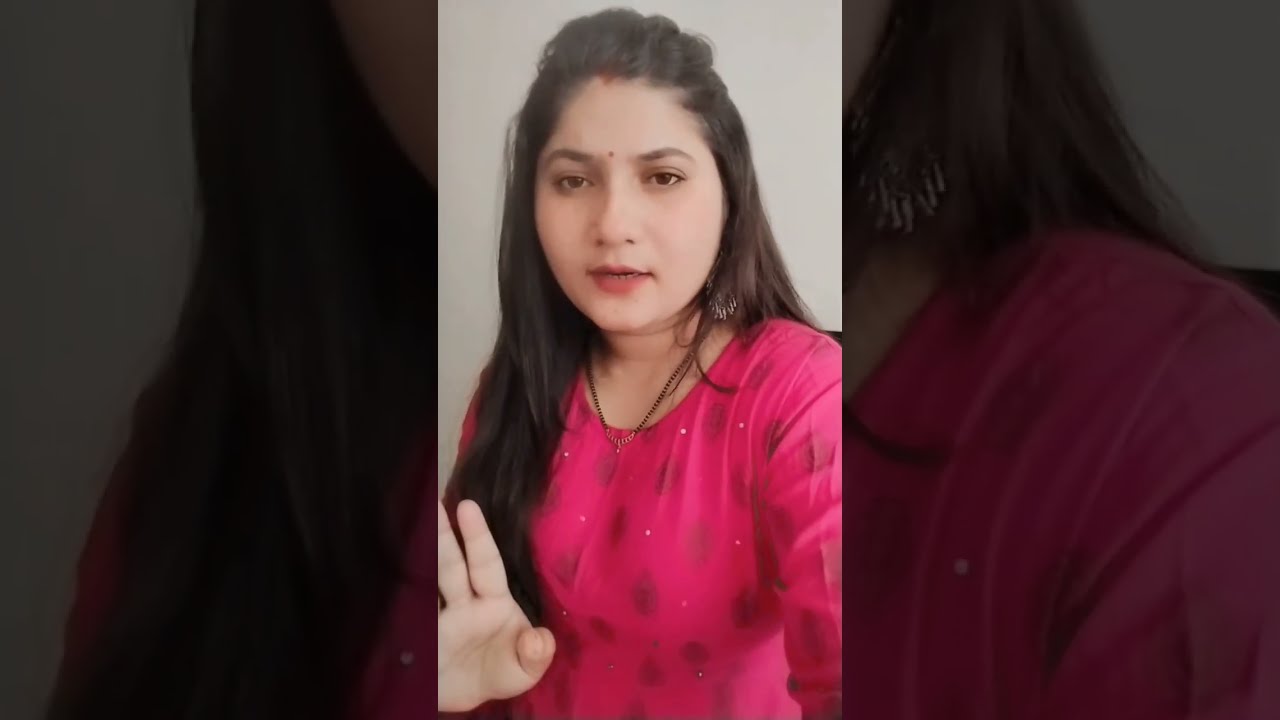This is a color photograph, seemingly taken in portrait mode from a smartphone, likely from a YouTube or TikTok video. The image features an Indian-looking woman in her late 20s to early 30s with long, black hair cascading below her chest. She is dressed in a pink or red shirt adorned with darker red spots or circular designs. She accessorizes with understated long earrings and a gold necklace. A distinguishing red dot is visible on her forehead between her eyebrows, and a small mole is situated just above her nose on the left. The woman, looking directly at the camera, has her mouth partially open as if captured mid-sentence. Additionally, her right hand is raised to the bottom left of the frame, palm facing the viewer with her thumb slightly bent inward. The backdrop is a solid off-white or light beige color, with darker, less illuminated details of the photo framing her on both the left and right sides.